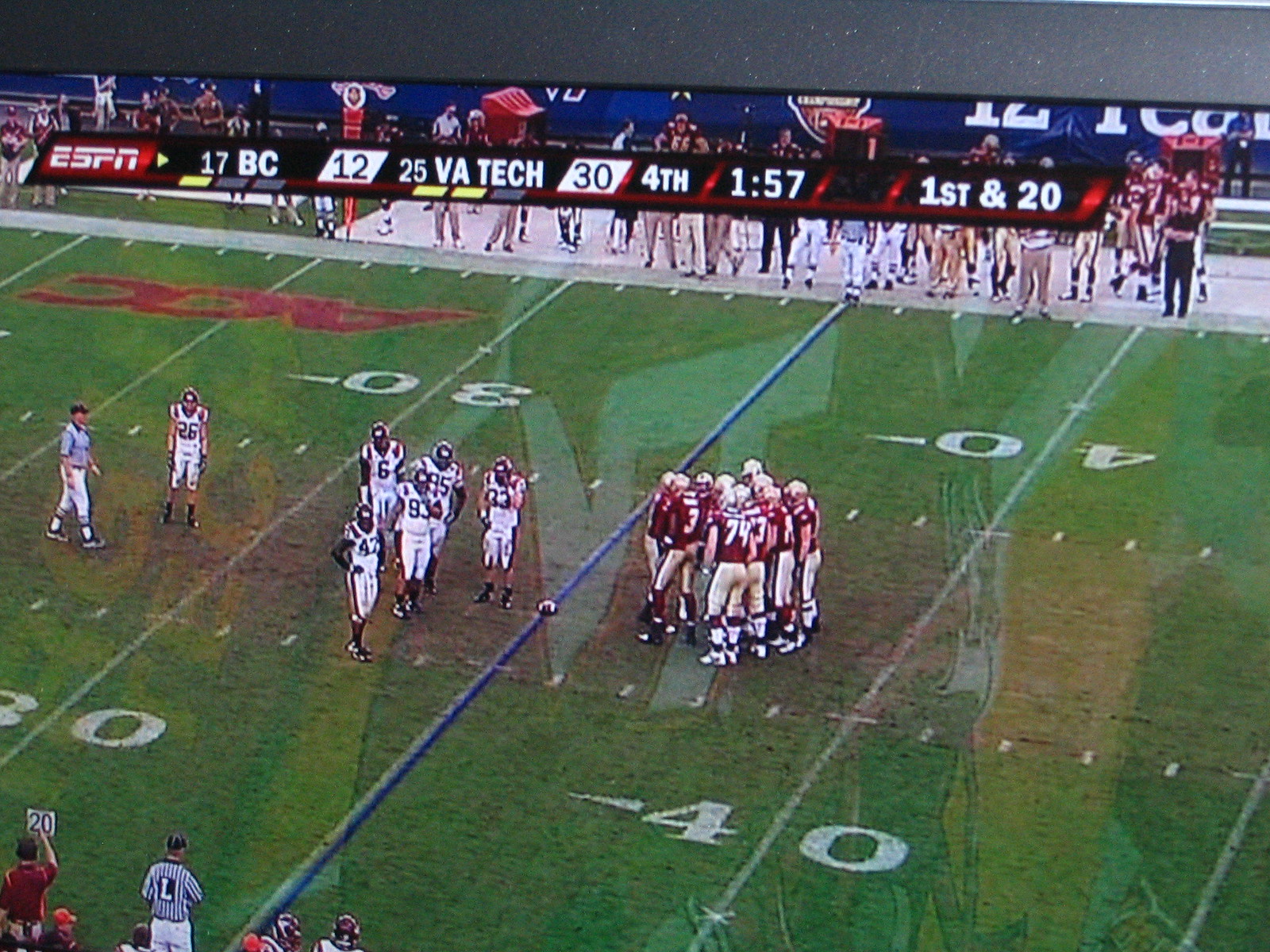This image captures a football game viewed from a unique angle that suggests it is being watched either through a high vantage point or from inside a special viewing box. The perspective is slightly elevated, looking down at the game from approximately a 30-degree angle, likely reinforcing the notion of a special glass box or a high seating position. The presence of reflections hints at the possibility of the game being viewed on a television screen, though the black bar with white specks at the top of the image, resembling a metal frame, makes this distinguishable element ambiguous.

The game appears to feature two teams: one team sports red tops paired with light golden or off-white pants, while the other team is dressed in mostly white uniforms accented with black and possibly a red stripe. The teams are dispersed between the 40-yard line and the 30-yard line. Confirming that the image is indeed a television display, there is a digital overlay bar at the top detailing pertinent game information: "ESPN, 17 BC, 12, 25 VA Tech, 34th, 157, 1st and 20."

In the background, a large crowd lines the sidelines, adding to the dynamic atmosphere. The angle of the shot means much of the crowd is observed at the top of the image. Positioned near the bottom left is a referee and a person holding a sign that reads "20." Surrounding them are the tops of heads belonging to other players.

On the field itself, the ACC logo is prominently displayed in red between the two teams. A blue line extends across the field, further dividing the two opposing groups of players, accentuating the tension and setup of the game.

This detailed observational scene provides a multidimensional representation of the football game, incorporating elements of both setting and action.